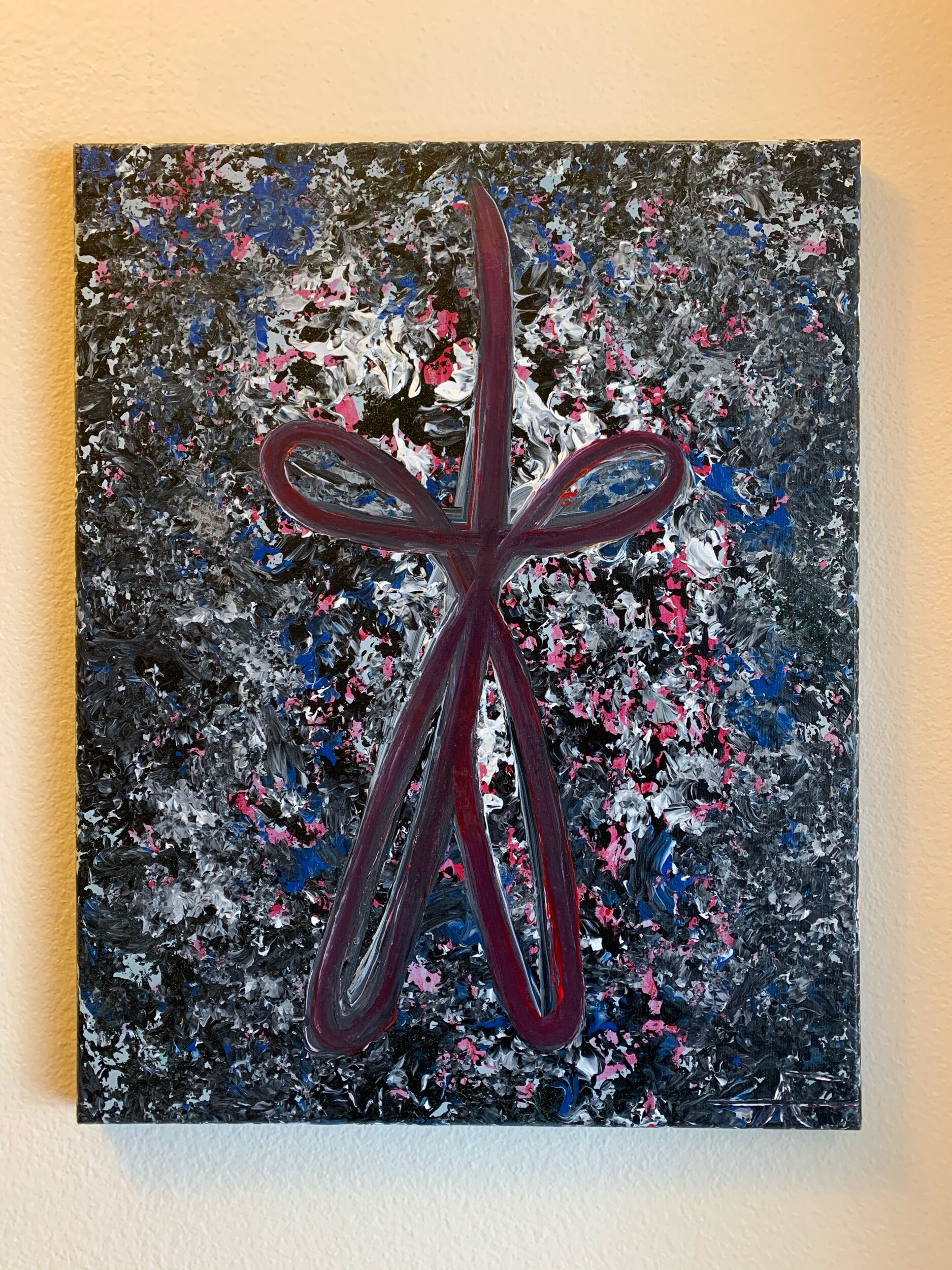The image features a photograph within a peach-colored rectangular frame, casting a yellow shadow to the left that fades into peach and transitioning to blue at the bottom right, blending into white and peach. The detailed background includes hues of black, dark gray, white, blues, and pinks, interspersed with blotchy patterns reminiscent of an abstract painting style, somewhat like Jackson Pollock's. Central to the photograph is a complex purple and red star or bow shape resembling a loopy peace sign, possibly drawn in lipstick or paint. The backdrop appears grainy and may depict a nature scene, possibly seaweed, foliage, or even a decorative carpet, indicating a vintage, pixelated quality suggestive of the 1970s or early 80s. The entire art piece is displayed on a beige cream-colored wall.